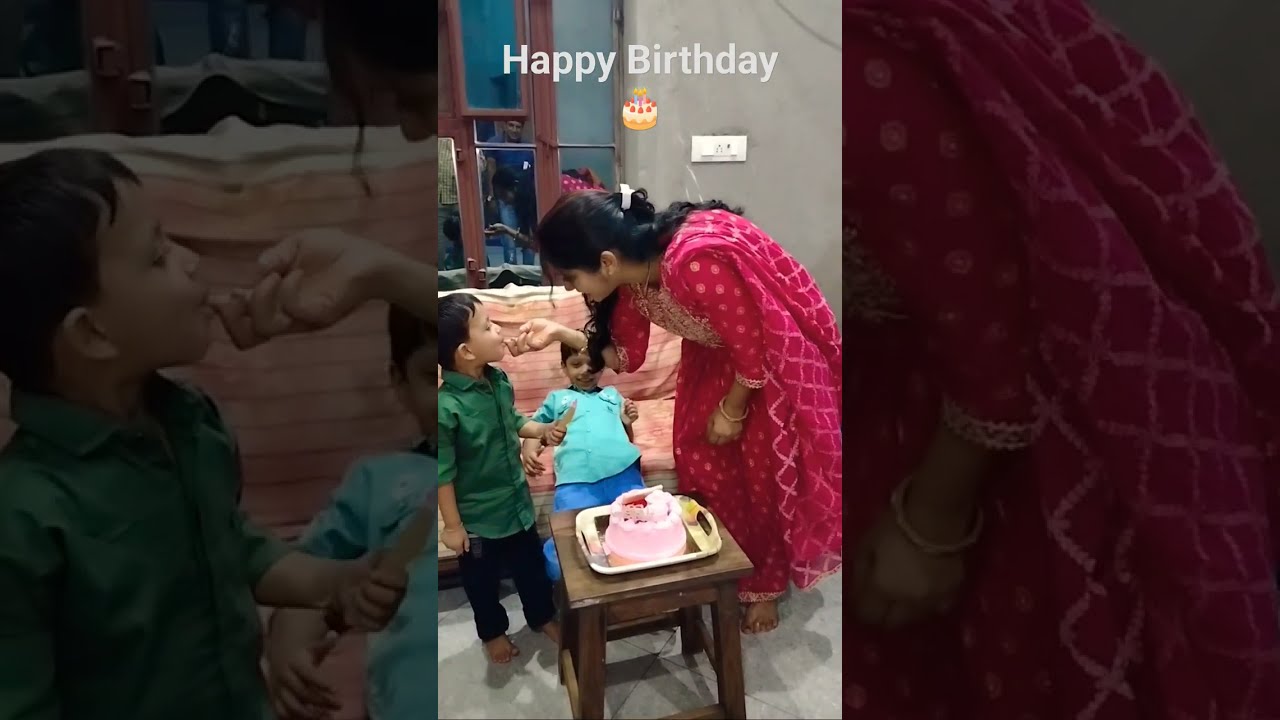Here's an image capturing a heartfelt moment from a birthday celebration. At the center of the scene is a woman, presumably the mother, with dark brown, flowing hair, dressed in a traditional, vibrant red and gold Indian gown. She has a bracelet on her left hand and is barefoot, standing on a white floor. She is gently feeding a piece of cake to a young boy, who seems to be around five years old. The boy is dressed in a clean green button-down shirt and dark pants, and is also barefoot.

Next to them, a slightly older child, dressed in a turquoise t-shirt and blue pants, reclines on a peach-red colored couch. The family is gathered around a small wooden table, atop which sits a birthday cake on a yellowish tray. The cake is decorated with pink frosting and appears to be a layered cake.

In the background, you can see a window with multiple panes, a round hanging lamp, and a wall adorned with a thermostat. The wall itself is a subtle gray. The words "Happy Birthday," in white capital letters, along with a birthday cake emoji, are prominently displayed at the top of the image, indicating the joyous occasion. The entire scene is framed as though taken from a cell phone, with broad bands of darkened portions on the left and right sides of the main photograph.